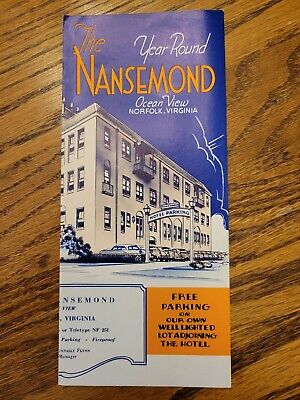The image features a vintage-looking brochure resting on a wooden tabletop. The brochure, titled "The Year-Round Nansmond Ocean View, Norfolk, Virginia," depicts a hand-drawn, cartoony rendition of a large, three-story, rectangular white building that resembles an apartment or hotel. This building is set against a backdrop of a dark blue sky with hand-drawn clouds. Below the building, a series of vintage cars from the 1950s and 60s are lined up in front, with an archway prominently displaying the hotel's name. The brochure also emphasizes amenities such as free parking on a well-lighted lot adjoining the hotel. Additional information is presented in smaller text boxes scattered across the cover, which include blue and orange text. The overall design is nostalgic, reminiscent of an era gone by, and suggests a fold-out format typical of brochures.